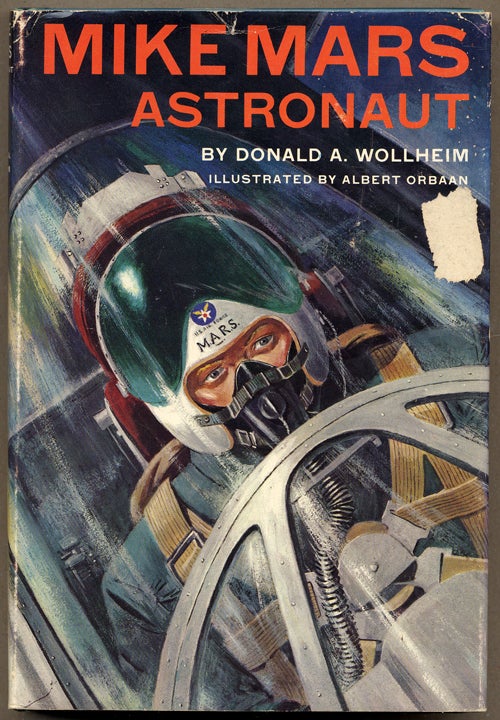The image depicts an old, tattered book cover with wrinkled and faded edges, resting on a brown surface. Across the top, in large red letters, it reads "Mike Mars," with "Astronaut" slightly smaller and directly beneath it. Below that, in white letters, it states, "By Donald A. Wollheim" and further down, "Illustrated by Albert Orban," though part of Orban’s name is obscured by a torn patch. The illustration on the cover features a man, presumably an astronaut, inside a rocket ship or jet cockpit. He is seated in a confined space, secured by brown suspenders and a large gray harness with front buckles. The astronaut is wearing a helmet with "Mars" emblazoned above his eyes, a visor he can pull down, and an oxygen mask connected by a black tube. The background shows a dark twilight sky with visible stars, adding to the outer space theme. The cockpit details include a silver frame and glass shield extending over and behind the astronaut.